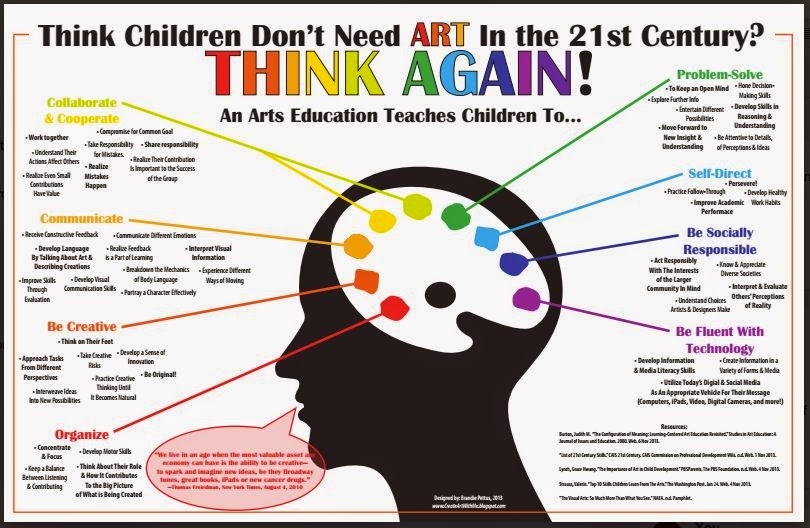The poster boldly proclaims, "Think children don't need art in the 21st century? Think again!" with "Think again" strikingly highlighted in rainbow colors (red, yellow, orange, green, blue, purple). Central to the poster is a blacked-out head with a white brain diagram, featuring various colored dots and arrows pointing outward. Each arrow is labeled to illustrate the multifaceted benefits of an art education, such as enhancing the abilities to collaborate and cooperate (yellow), communicate (orange), be creative (dark orange), organize (red), problem solve (green), self-direct (blue), be socially responsible (blue), and be fluent with technology (purple). This intricate visual underscores the comprehensive intellectual and social skills that children gain through art education. There's also a small, unreadable sign emerging from the person's mouth. The entire design emphasizes the critical, multi-dimensional value of incorporating art into modern education.